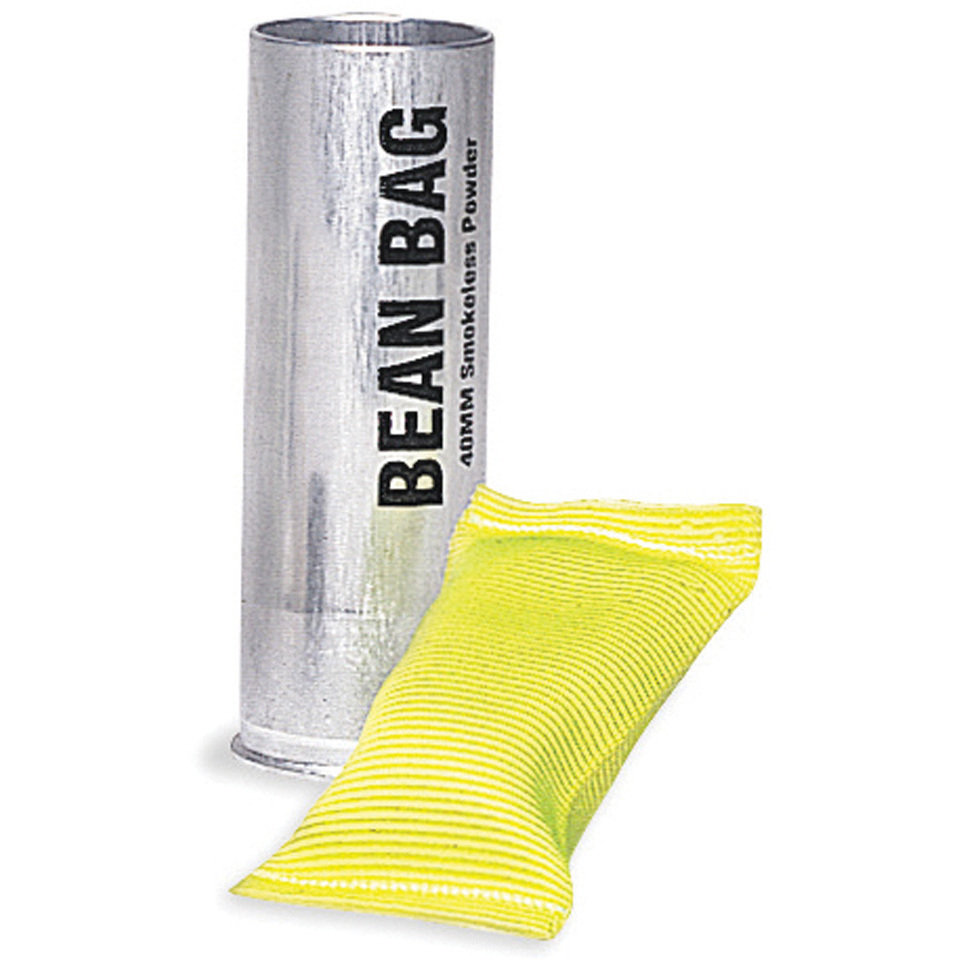The image showcases a promotional product typically found on an e-commerce website, featuring two distinct elements against a pure white background. On the left stands a silver cylindrical shell casing with an open circular top, displaying bold black text that reads "BEAN BAG." Beneath this, smaller text specifies "40mm Smoke-Free, Smokeless Powder." Positioned to the right of the canister lies the actual bean bag, characterized by its long rectangular shape, shaded mainly in yellow and lined with both thin and slightly wider black lines. The bean bag appears to be a few inches thick and about three to four inches in length, giving an impression of being filled with some material. This niche product, likely designed for specialized use, combines the shell casing and the bean bag in a manner that suggests the bean bag could be loaded into the casing to be fired or deployed, rather than being a typical supermarket item.